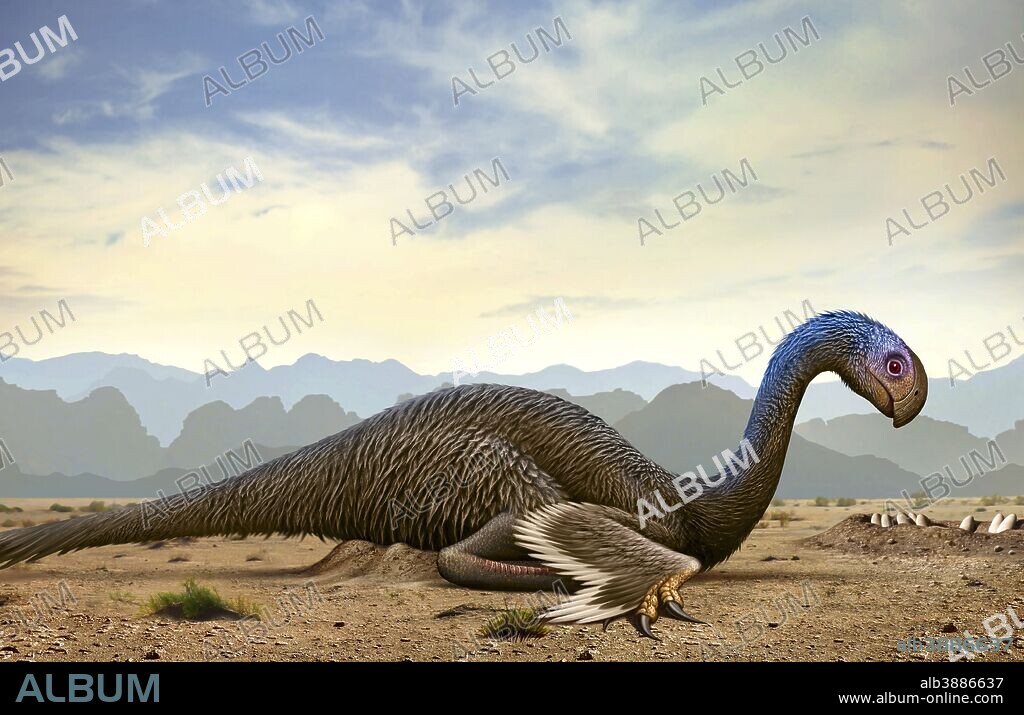This detailed image captures a fantastical or prehistoric large bird with a striking blue head and a curved beak, laying on a compacted dirt ground. Its small wings rest by its sides, and it has a distinctive long tail. The scene is set in what appears to be a desert environment with a hazy outline of brown and blue mountains in the background under a clouded blue sky, tinged with light brown or yellow hues. Notably, in the right-hand corner of the image, there is a pothole containing nine eggs. The bottom corners of the image feature the website URL "ALB3886637www.album-online.com" and the word "album," which is repeated across the entirety of the picture, giving it a distinctive watermark.